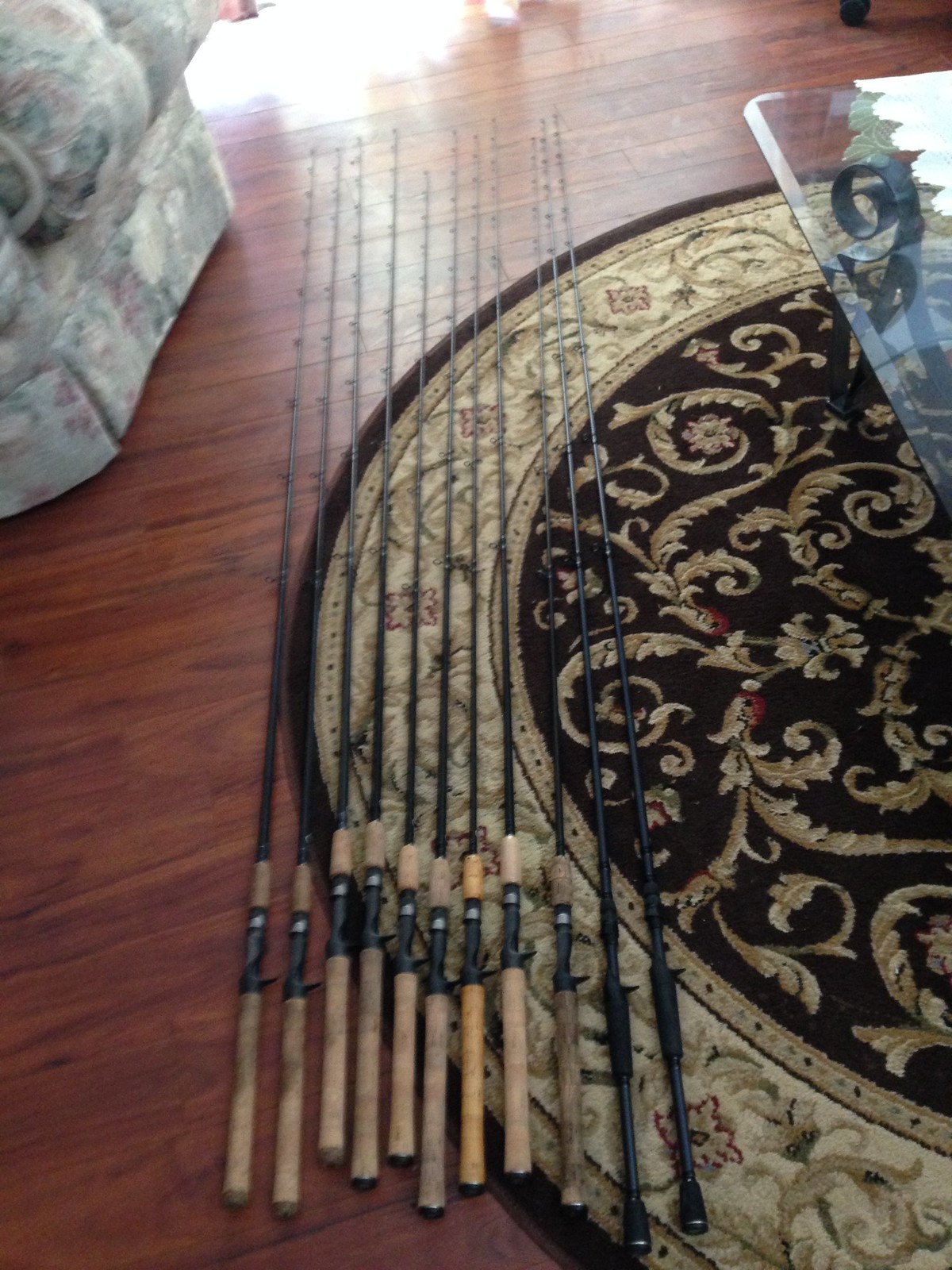The image depicts around a dozen fishing rods neatly laid out on the medium brown wooden floor of a home. The rods are aligned parallel to each other, with their handles at the bottom of the image and their tips pointing toward the top. Most of the rods feature tan cork handles, except for the two on the far right which have black handles, and one with a unique yellow handle in the middle. They partly rest on a circular rug with a multifaceted design, featuring an inner circle in black adorned with goldish-brown, dragon-like patterns, and an outer circle bordered in brown with a cream background and red and pink floral motifs. In the upper left, a floral-patterned armchair is visible, though blurry, while the upper right shows part of a glass-top table with a black metal base.